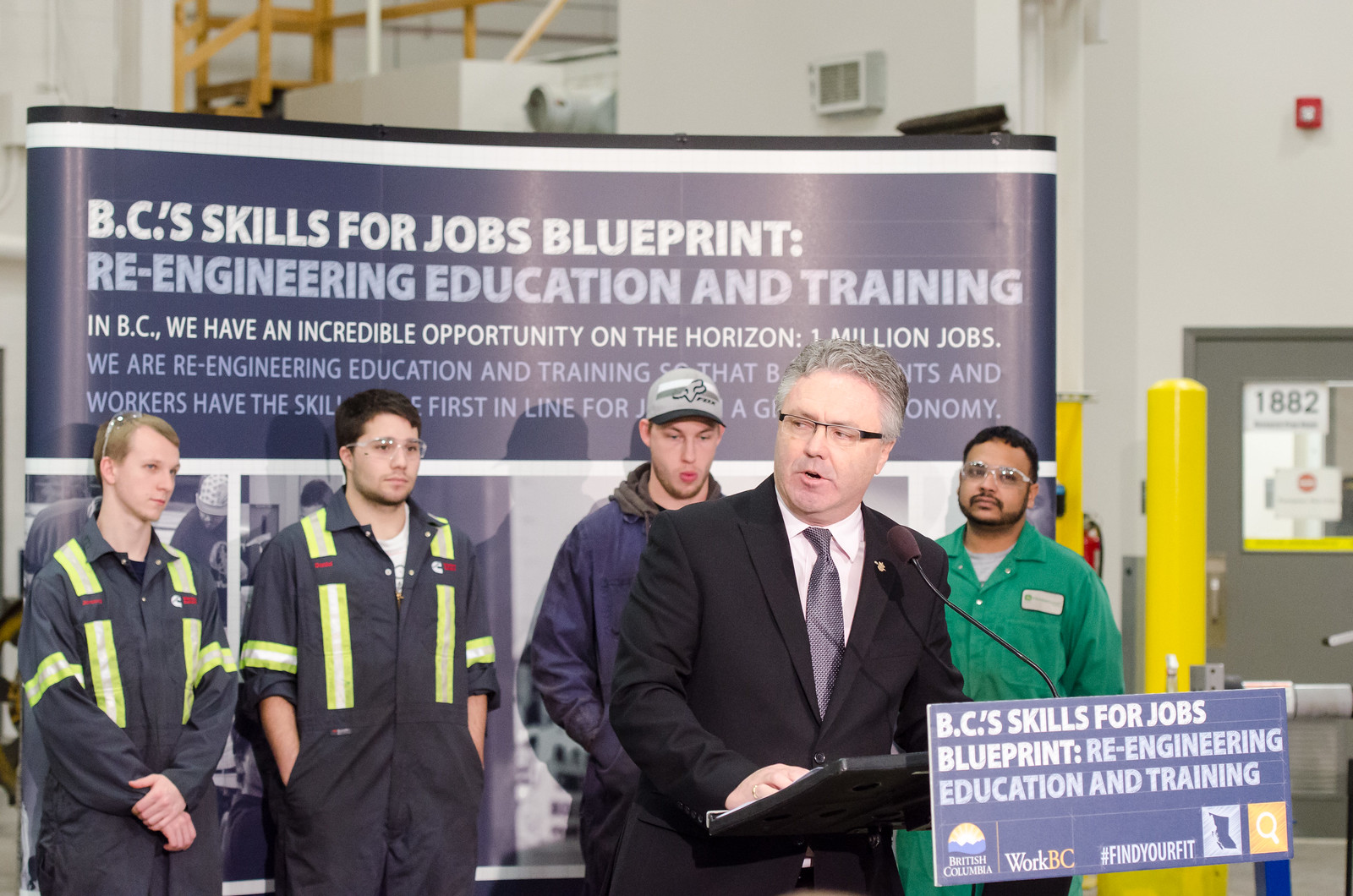The image depicts a distinguished man with gray hair and glasses, clad in a black suit, white shirt, and gray tie, addressing an audience from a podium. The podium displays a sign that reads "BC Skills for Jobs Blueprint: Re-engineering Education and Training." The backdrop reiterates the same message, emphasizing a forward-looking plan for creating opportunities and equipping workers with essential skills in British Columbia, highlighted by distinct blue and white typography. Surrounding the speaker are four men in various uniforms: two dressed as firefighters in orange safety gear, one in a green button-down shirt with matching pants, and another in a gray hoodie and cap. The setting is a room characterized by white walls and yellow pillars, denoting a formal event focused on labor and training initiatives within the region.